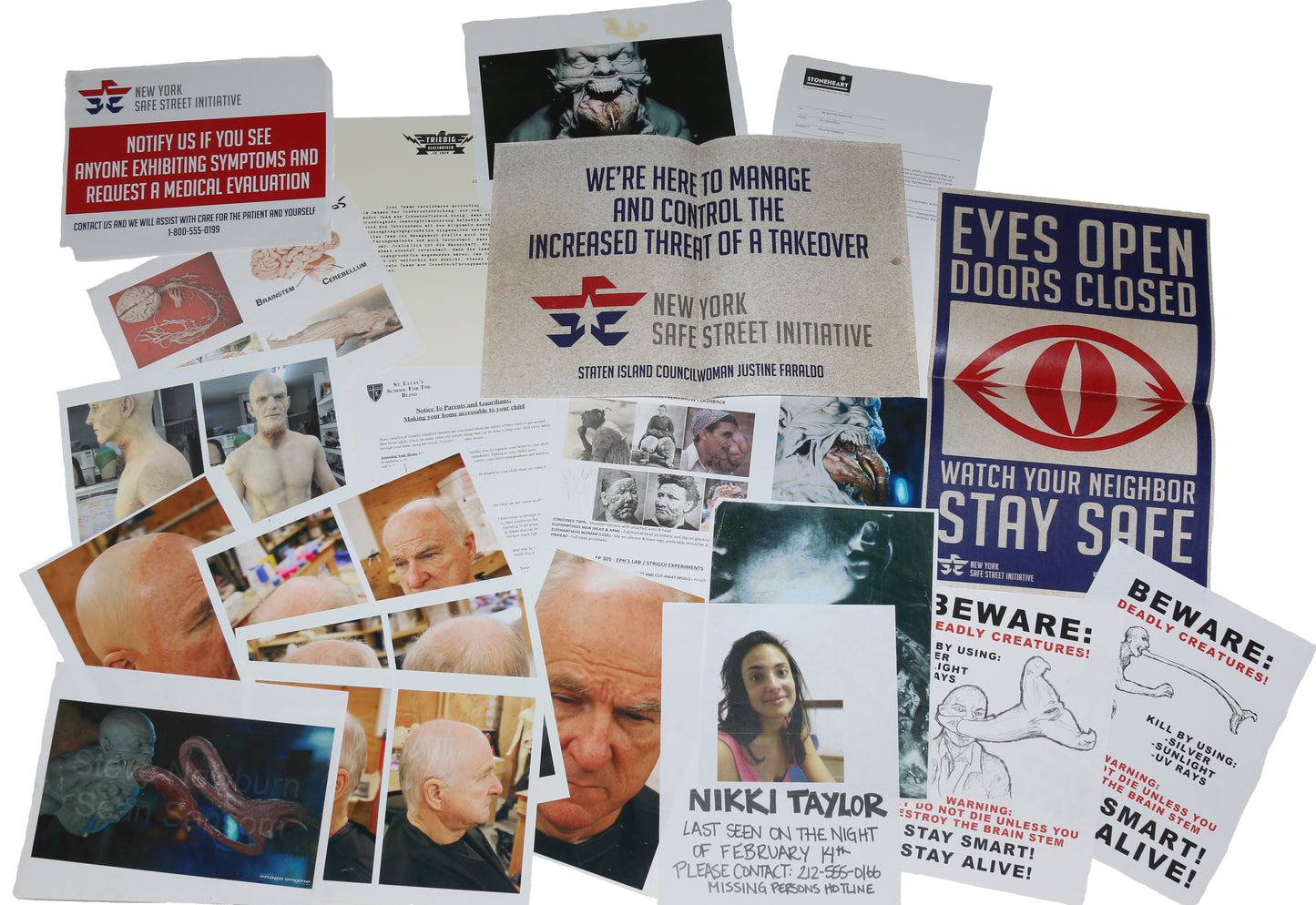This horizontal, rectangular image is an eclectic composition of posters, stickers, and photographs, arranged for partial readability. Dominating the upper left is a large blue poster featuring an eye with a red pupil and the foreboding text: "Eyes Open, Doors Closed. Watch Your Neighbor, Stay Safe." Below it, there are two white posters sharing the slogan: "Stay Smart, Stay Alive." To the left of these, a poster featuring Nicky Taylor can be seen. 

In the center, another sticker sternly states: "We're here to manage and control the increased threat of a takeover," followed by "New York Safe Street Initiative" in gray below. The bottom left highlights a series of color snapshots showing a man getting his head shaved at a barbershop, while the bottom right displays a woman named Nikki Taylor on a white sticker, labeled with her last known location and contact information for sighting reports. The collage combines sci-fi themes, ominous messages, and vintage aesthetics, woven together in a mixture of color photos and black-and-white line art with spot coloring, suggesting a visual reference for a potential sci-fi narrative or film.